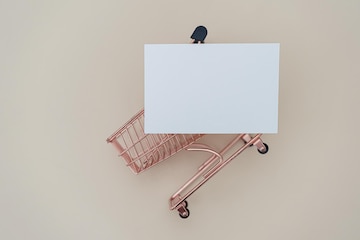The image features a small, toy-sized shopping cart, predominantly colored in a rosy bronze or copper hue. The cart is laid on its side with the front part facing down and towards the bottom left of the frame, showcasing its finely detailed construction. Black wheels at the bottom and a black handle peeking out at the top are clearly visible. The background is an off-white or light gray, creating a neutral setting that contrasts with the cart’s vibrant color. A large, plain white rectangular piece of paper or possibly a digitally-altered white rectangle obscures much of the cart, covering its handles and a significant portion of the basket. The exposed parts include the front section of the basket, the bars connecting it to the rest of the frame, and part of the wheels, giving the viewer a glimpse of its intended design and small, artistic details. The overall composition suggests a whimsical yet artistic portrayal of an everyday object, emphasizing its miniature scale and distinctive coloring.